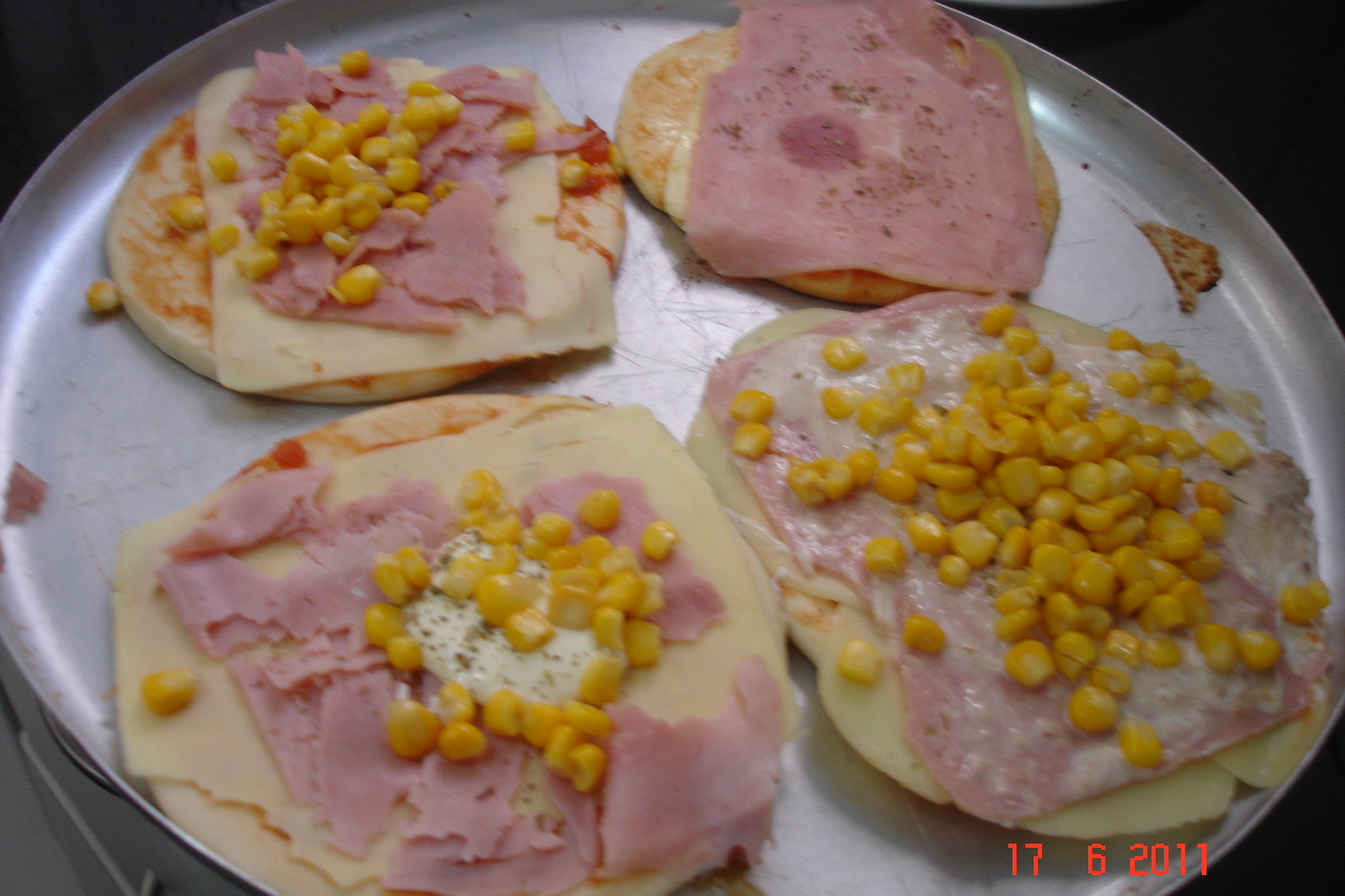This image is a color photograph of a homemade food dish taken on June 17, 2011, as indicated by a red date stamp in the bottom right corner. The food is arranged on a scratched, round aluminum tray reminiscent of a pizza pan. There are four open-faced concoctions, possibly small pizzas or bagel halves. Each base appears to be a toasted English muffin or a piece of bagel, spread with a red sauce, likely ketchup or pizza sauce. They are topped with square slices of white cheese, such as mozzarella, or possibly provolone.

Various pieces of deli ham—some sliced, some torn—are added on top. Three of the four open-faced sandwiches are heavily garnished with yellow corn kernels. One of them may also have a dollop of white sauce, perhaps mayonnaise or something of similar consistency, sprinkled with green specks which might be herbs or pepper. The fourth item, located at the top right, is distinctive in that it has only ham and cheese, and lacks the corn and white sauce seen on the others. The overall presentation looks homemade and rustic, with bits of cheese and corn scattered on the reflective but dull metal surface of the tray. The image is lit from above, casting light on the textured food and tray.